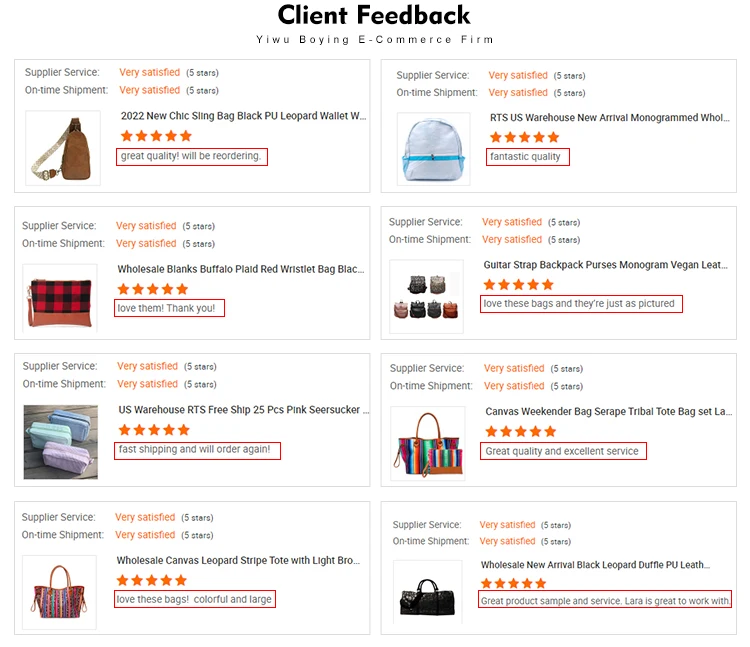This is a detailed snapshot of a shopping website focused on client feedback and product offerings. At the top of the page, in bold black text, it prominently displays the header "Client Feedback." Directly beneath this title, the website name is featured: "YIWU Buying E-Commerce Firm." 

Below this, the site showcases eight different items currently available for purchase, each accompanied by a small image of the product, a star rating, and a title. All the displayed items are various types of bags: 

1. Four of the items are stylish purses designed for everyday use.
2. One is a practical yet fashionable backpack, ideal for carrying essentials securely.
3. Another item is a set of small makeup bags, perfect for organizing cosmetics.
4. Lastly, there is a unique monogrammed backpack purse, combining the versatility of a backpack with the elegance of a purse.

Each product is arranged in a neat and visually appealing manner, highlighting the variety and quality of the bags offered by the YIWU Buying E-Commerce Firm.